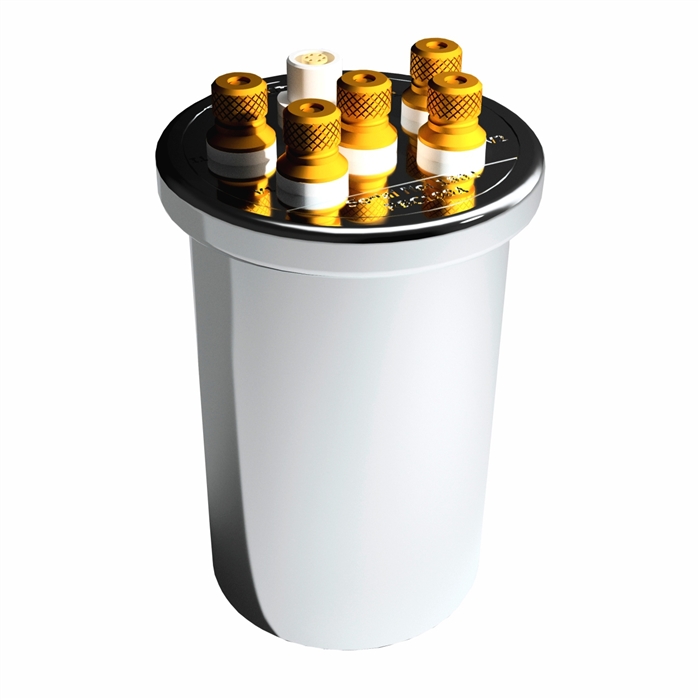The image depicts a cylindrical electronic device with a white body, resembling an upside-down bucket or cup. At the top, the device features a silver lid adorned with five golden knobs, each with a white base, and a crisscross pattern along with small holes. Additionally, there is one extra white knob situated behind the golden ones. The knobs are placed on a silver surface at the top of the device. Some text is visible, scribbled at the bottom part of the silver surface. The entire setup casts a shadow on the left side, and the background of the image is plain white.